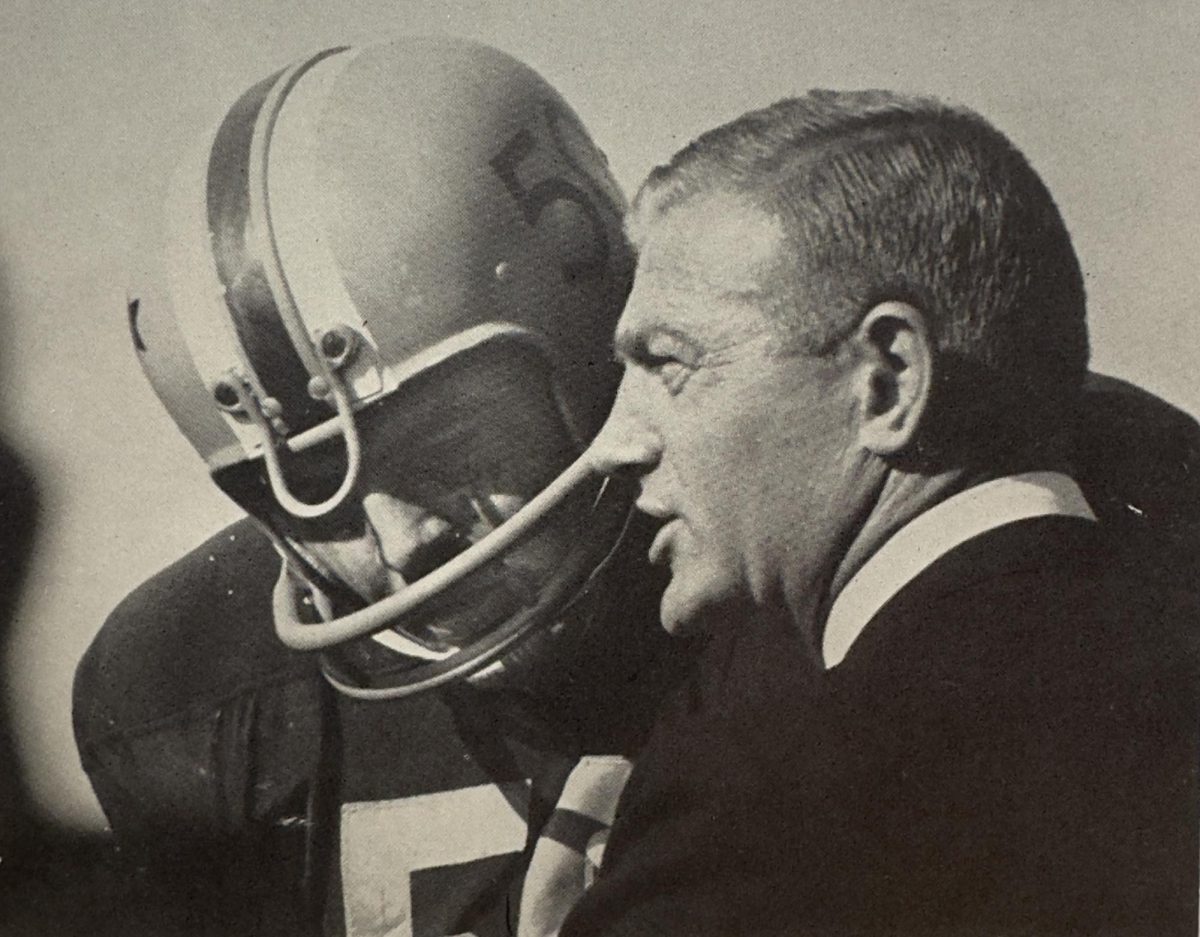This black-and-white photograph captures a poignant moment from the 1930s or 1940s between legendary football coach Dick Butkus and a football player wearing the number 50. The player, whose head is slightly tilted downwards to listen closely, dons an old-school helmet marked with three distinctive stripes—two white flanking a dark center stripe—and a rudimentary face mask with two wide gray bars creating a mouth-like appearance. His uniform is dark, with the visible part of the jersey showing a large white "50." On the other hand, Coach Butkus, slightly older with noticeable wrinkles and squinting eyes, stands in a black suit jacket and a heavily starched white collared shirt. His body is turned away from the camera, with his head in profile, as he gazes into the distance while speaking into the player's ear. The backdrop features a gray sky, amplifying the timeless feel of this powerful exchange.